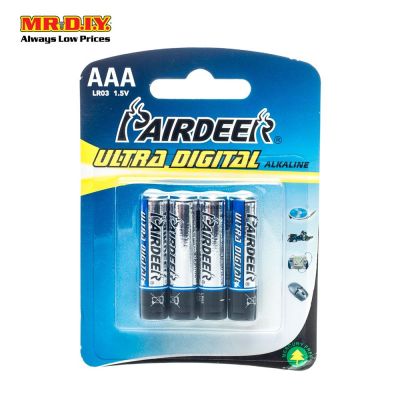This product image features a package of AAA batteries set against a white background. The packaging showcases a vibrant and eye-catching design with multiple elements. In the upper left corner, the brand name "Mr. Dot DIY" is prominently displayed in playful red bubble font, accompanied by the tagline "Always Low Prices" in an understated black font just below it.

The package itself is attached to a sturdy cardboard backing, which has a unique cube shape with slight rounding at the top. There is an oval-shaped cutout at the top center, designed for hanging on retail display hooks. The cardboard backing exhibits a blue gradient, transitioning from a dark shade at the top to a lighter blue in the lower right corner.

At the top of the packaging, in white font, the product type "AAA" is clearly indicated. Directly beneath, the brand name "Pear Deer" is written in bold black font. Below the brand name, the product's attributes are listed: "Ultra Digital" in bright yellow font followed by "Alkaline" in black font.

Encased in a clear plastic blister at the bottom of the cardboard backing are four AAA batteries, securely held in place. The transparent plastic allows the batteries to be easily viewed, ensuring the consumer can see the product clearly.

Overall, the packaging effectively combines functionality with a striking visual presentation, ensuring it stands out on the shelves.